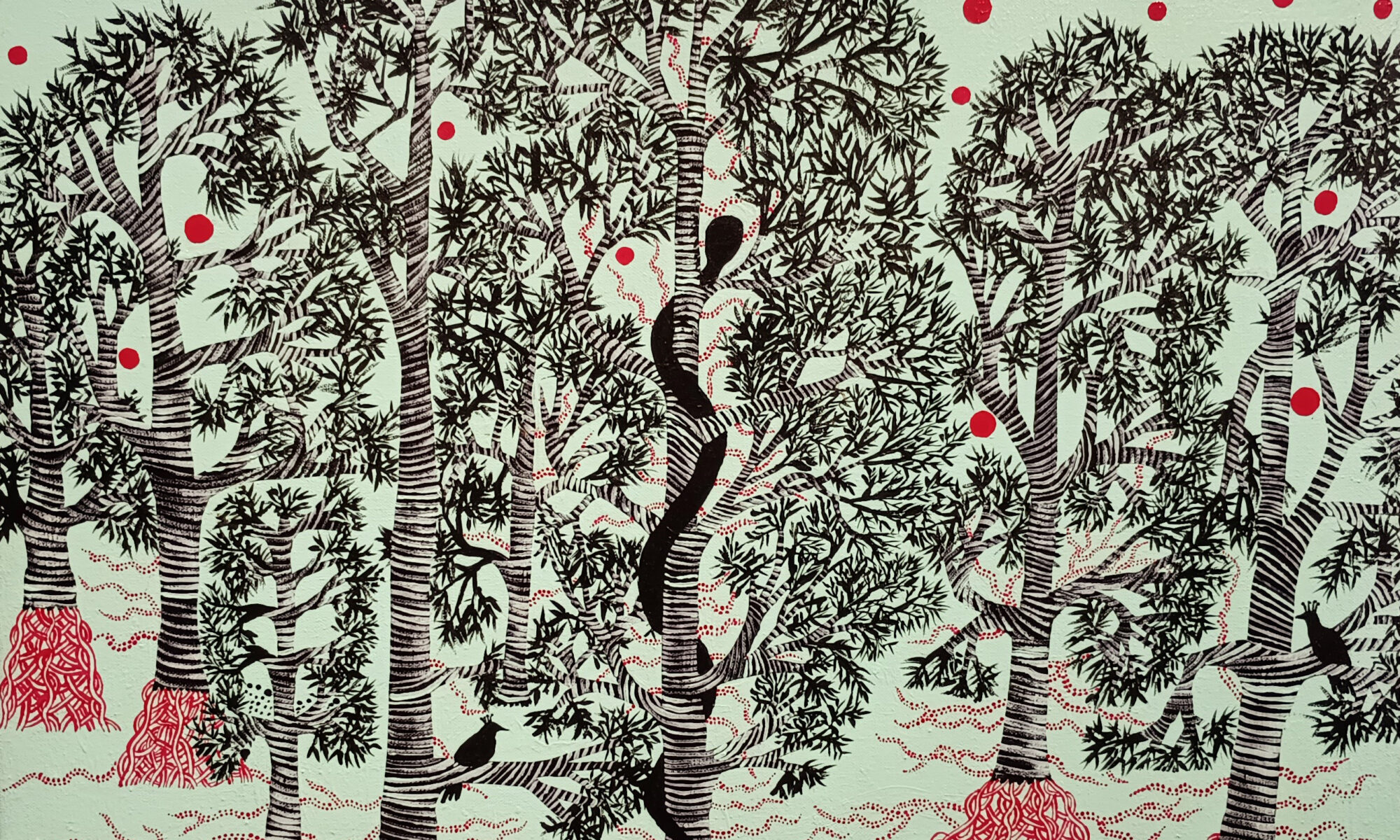The artwork depicts a forest scene with a light mint green background. Intricately illustrated, the trees are drawn using black ink, their trunks spiraled with horizontal lines. The trees appear almost cartoonish and evoke a Japanese-style aesthetic. The foliage is marked by numerous small, red circular objects, reminiscent of apples. At the base of three prominent trees, red formations—potentially representing roots—branch out and spread across the ground. A black snake coils around the trunk of the central tree, introducing a possible reimagining of the Garden of Eden. Adding to the forest ambiance, a blackbird perches among the branches while a silhouette of another bird appears on the ground. The detailed black-and-white elements against the mint green backdrop create a visually striking and thought-provoking piece.